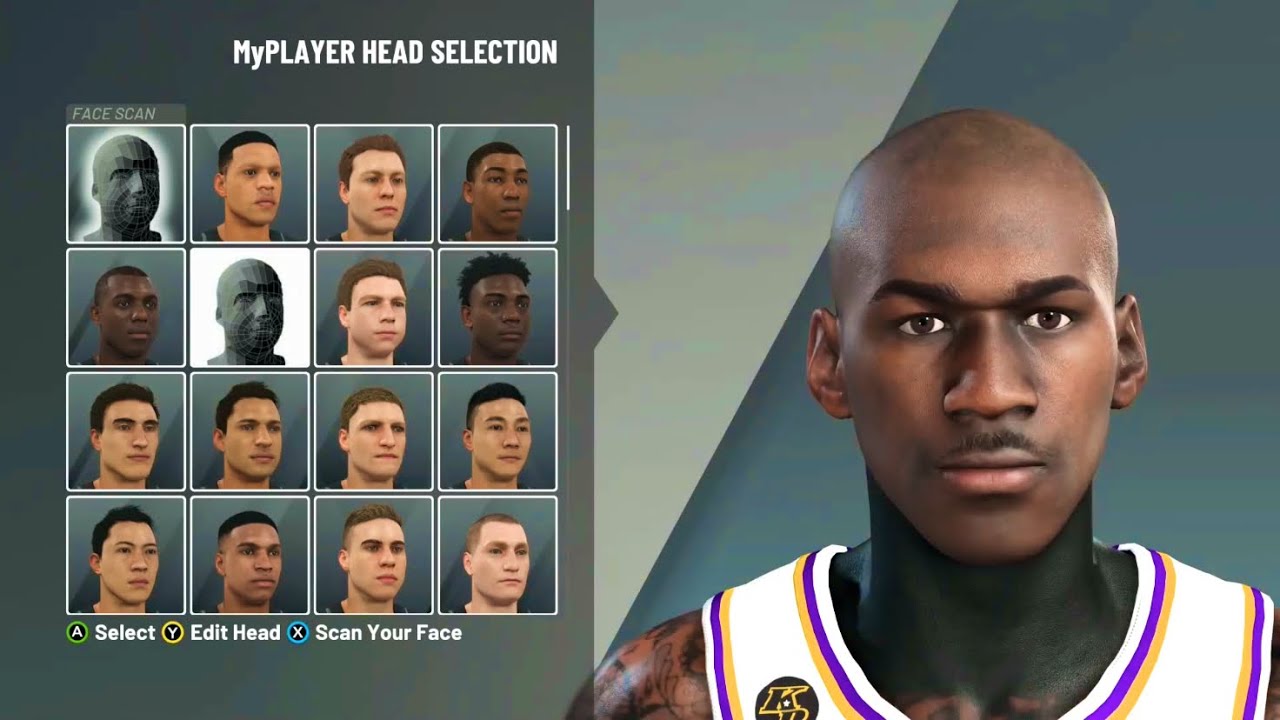A detailed window from a sports video game, likely a basketball game, is displayed. The interface consists of two main sections. On the left, a grid of 16 customization options (four rows and four columns) allows players to adjust their character’s appearance. Each character head in the grid is defined by a white outline against a dark gray background, showcasing various races and hair colors, typically representing individuals in their late 20s to early 30s. At the top of this section, in white letters, is the heading "My Player Head Selection." Beneath it, the options "Select," "Edit Head," and "Scan Your Face" are listed.

On the right side of the screen, the main character, a young bald male, is depicted. He has numerous tattoos on his left shoulder and is set against a mostly dark gray-green background which transitions to a lighter gray in the upper left corner. He is wearing a white jersey with pink and yellow stripes, featuring a distinct dark circular logo on the right shoulder, which contains a prominent "K."